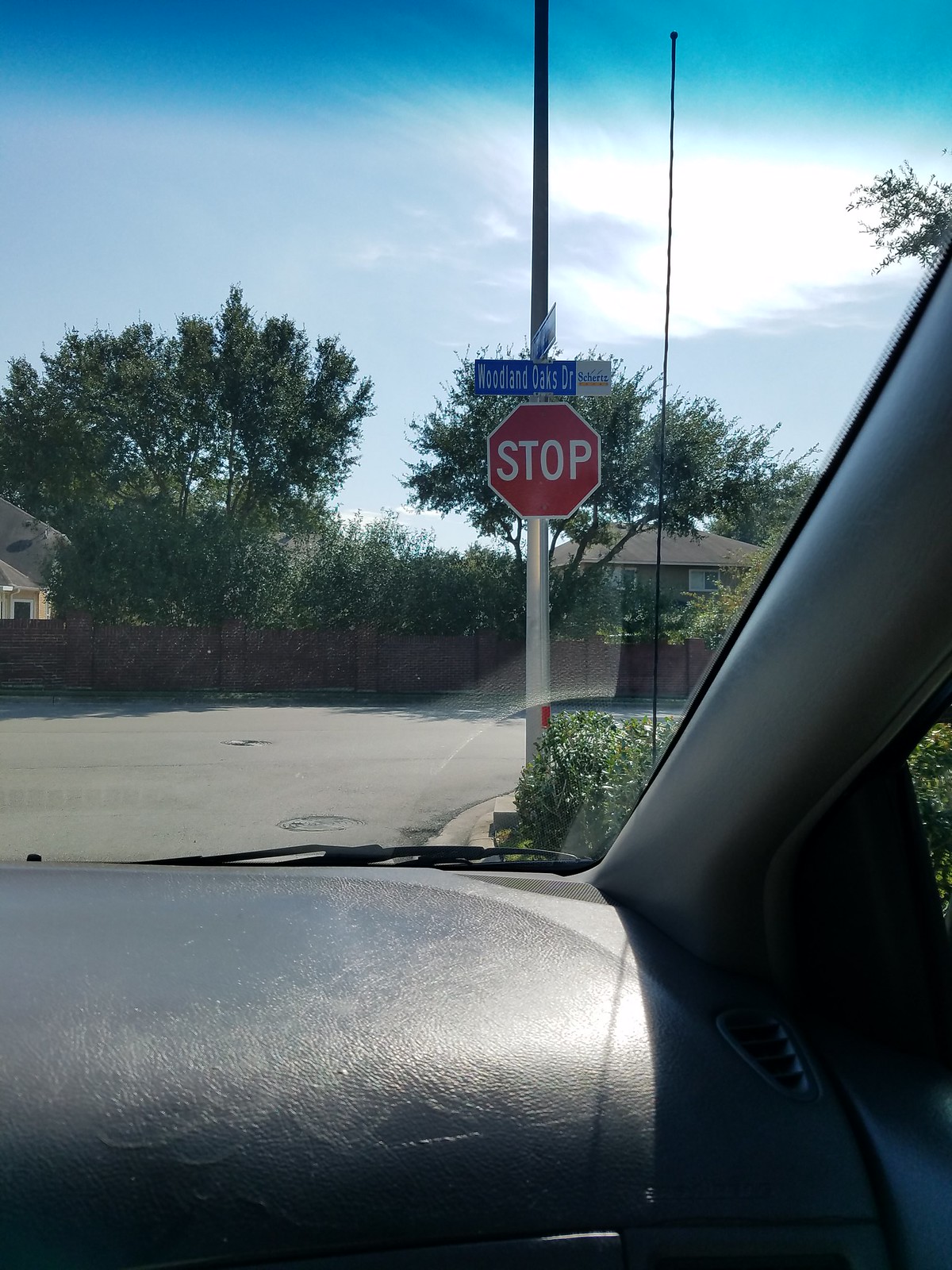This color photograph captures the view from inside a dark grey vehicle, positioned slightly before a stop sign. The stop sign, a standard red hexagon with "STOP" written in white, dominates the center of the image, located near the upper edge. Directly above it, a blue rectangular street sign with white text reads "Woodland Oaks Drive." Both signs are mounted on a silver metal pole. 

In the foreground, the car's dashboard is visible, featuring black leather and grey material, with a small black vent at the bottom right. The vehicle's bonnet, reflecting sunlight, is also seen through the front windscreen. Below the stop sign, a patch of grey ground can be observed, surrounded by green foliage and large trees. In the far background, beyond the trees, a house with a grey roof is partly visible. The sky is predominantly clouded grey with a section in the upper right corner showing clearer white and blue hues. The scene suggests it is a partly cloudy day.